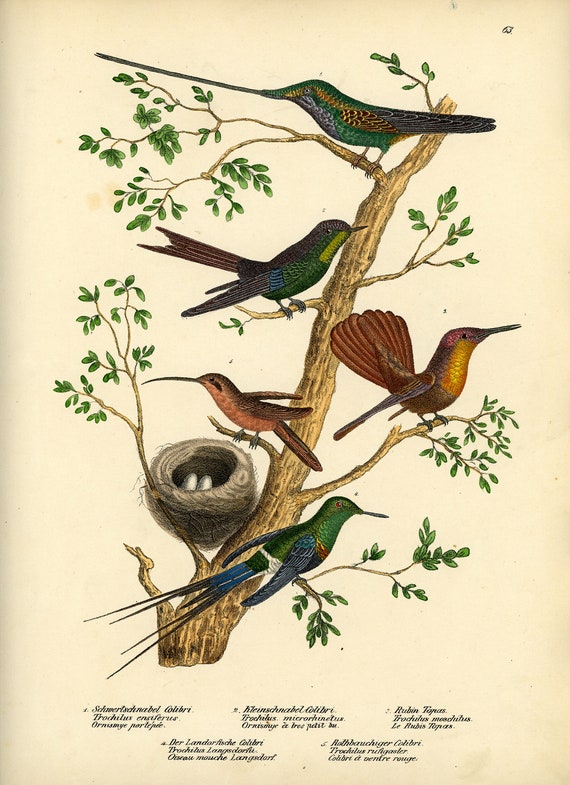The scanned image depicts an intricately detailed drawing of various bird species perched on a tree with abundant green leaves. Centered in the illustration is a nest containing two eggs. 

At the top of the tree, a bird with green, yellow, and black feathers featuring a long thin beak is perched. This bird is suggestive of a woodpecker or a hummingbird due to its distinctive characteristics. Below it, another bird with a green body, blue wings, and long tail feathers can be observed.

Moving rightward from the top, a bird with a red underbelly and orange wings can be seen, accompanied by a smaller beaked bird that showcases a combination of green, blue, and brown with a brown tail feather. Toward the middle left, a bird with a green underbelly and black wings is depicted. Additionally, one of the birds, with primarily brown feathers adorned by a hint of gold and yellow around its neck and chest, perches above the nest.

The text beneath the illustration is written in cursive and includes various Latin, French, and German phrases, such as "SCHWER," "Caligre, Trachulis," and "KLEINSCHNABEL." These labels presumably classify the birds species and provide related information, although they become increasingly difficult to decipher due to the small, out-of-focus print.

This image captures the natural beauty of these birds in a lush, leafy setting, depicted through precise and vibrant pencil drawings.